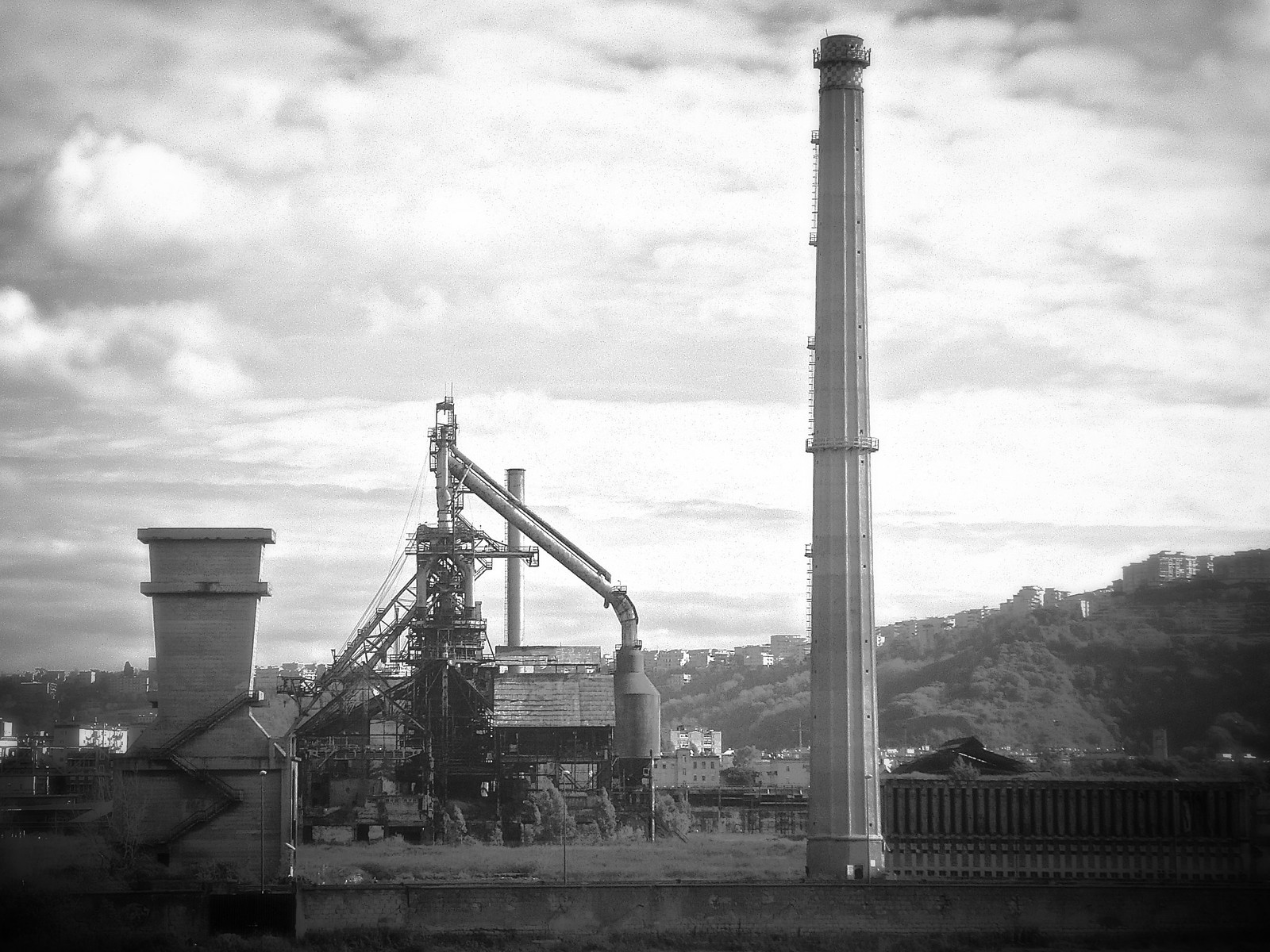The black-and-white photograph showcases an older industrial mill nestled in a valley, framed by mountains and rolling hills. Dominating the scene is a tall, narrow tower with a ladder attached to its side, leading to a small balcony or railing at the top – possibly serving as a lookout or having some mechanical function. To the left of this towering structure, the mill's intricate machinery is visible, featuring a chute connecting to a broader silo and additional scaffolding that merges into a building portion. The mill appears aged, emphasizing historical significance rather than modern industrial prowess. The bottom left of the image includes a brick structure, which might be a chimney, and nearby pipes. In the foreground are trees, houses, and a hilly treetop area, while the background is dominated by a cloudy, gray sky. The scene is devoid of people or text, adding to the timeless, contemplative feel of the photograph.